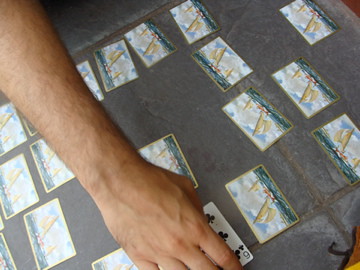In the image, a man’s hand is poised over a scattered deck of playing cards on a tabletop or possibly a tile floor. A single card, the six of clubs, lies face-up amidst the haphazardly spread cards, revealing its black clubs and white background. The other cards, while not uniformly arranged, show hints of blue and gold, featuring various images, one resembling a sailboat. Despite these splashes of color, the overall scene lacks vibrancy. There is no additional text or lettering present in the image, just the man's hand and the disarrayed cards on the stone-like surface.